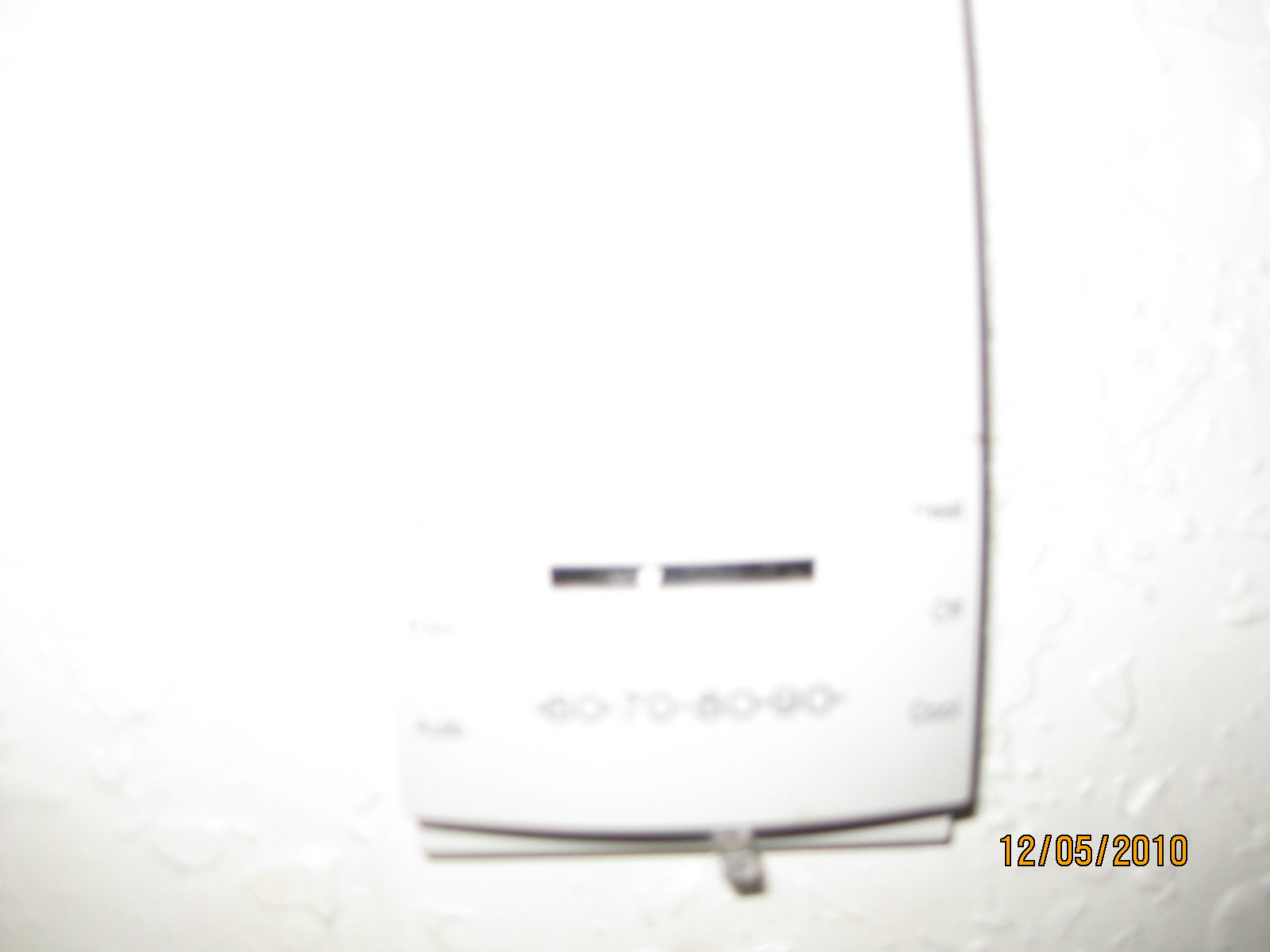This photograph, dated December 5, 2010 (as indicated by the yellow date stamp in the bottom right corner), features a close-up view of an old-style thermostat mounted on a white wall. The wall exhibits an irregular, somewhat dirty texture reminiscent of aged stone. Dominating the image, the thermostat displays a lever at the bottom, used to adjust the temperature. Though extremely blurry, the Fahrenheit scale, marked at increments of 60, 70, 80, and 90, is discernible. To the right of the lever, faint labels for "cool," "off," and possibly "heat" are noted, while the left side has two completely unreadable settings. A significant portion of the image is obscured by a harsh white glare, likely from a nearby light source or the camera’s flash, further distorting any additional details. The excessive brightness adds a mysterious quality to the photograph, creating an intriguing, albeit challenging, visual experience.